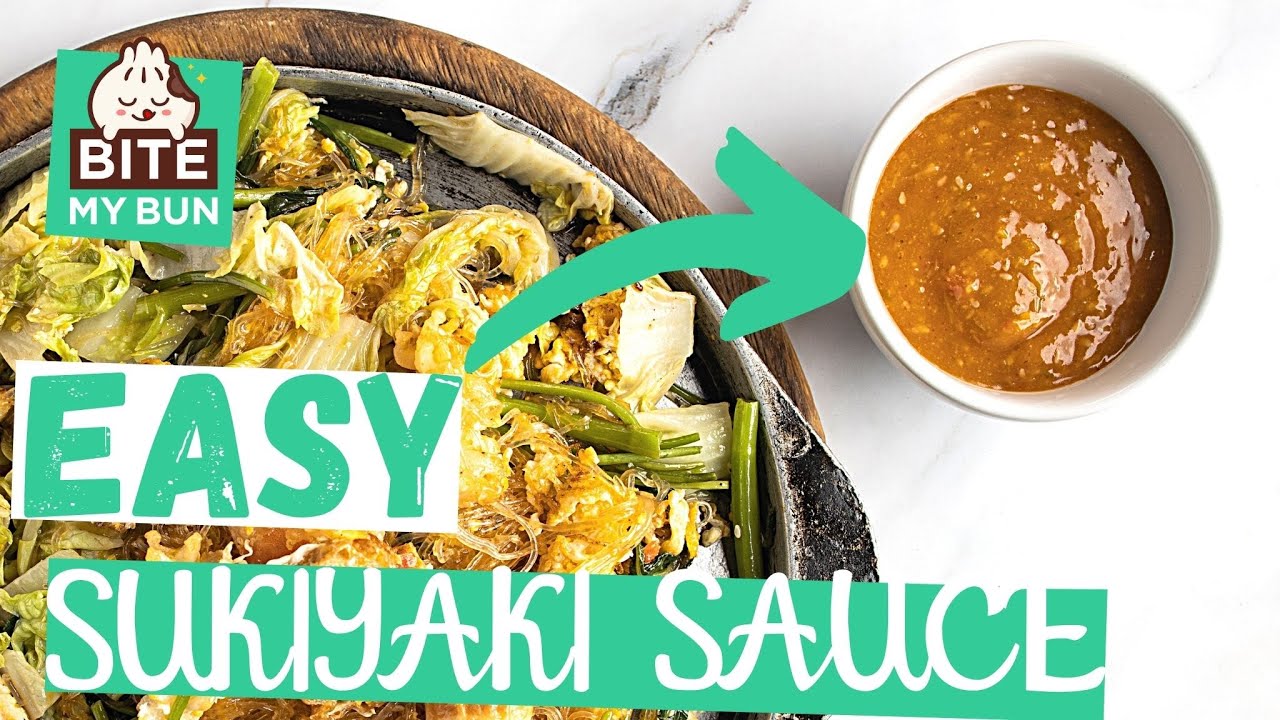The image appears to be an advertisement that promotes an "Easy Sukiyaki Sauce." In the upper left corner, there's a cartoon figure contained within a square box, with text that reads "Bite My Bun." Below this, there is a label in a greenish-blue color on a white background that says "Easy Sukiyaki Sauce." An arrow from this text points to a small white bowl containing a brownish, grainy sauce with seeds, positioned in the upper right corner. Toward the middle to the left, there's a wooden bowl with a stainless steel insert filled with a variety of cooked vegetables, likely including cabbage, celery, and possibly asparagus or bok choy. The bowl rests on a white table, adding to the clean, appealing presentation.